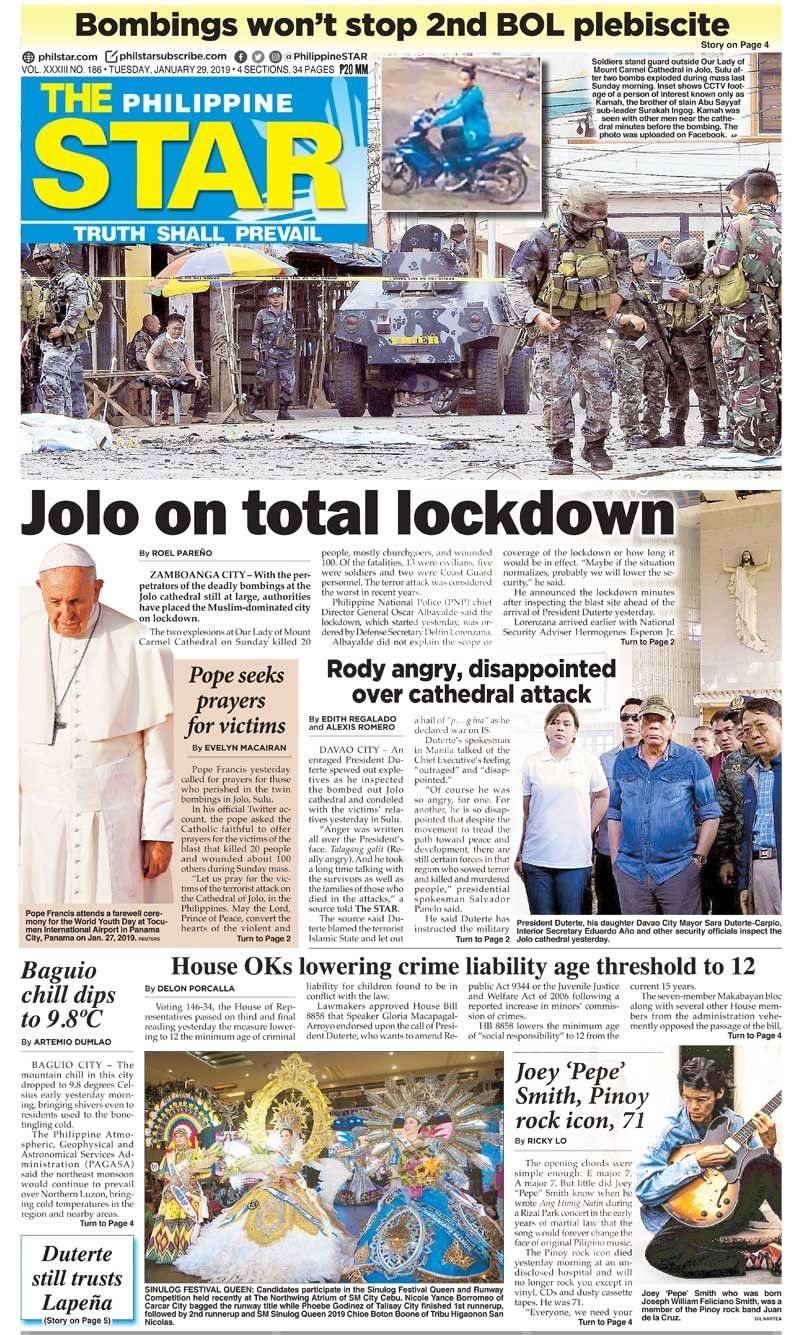A detailed image description of an online version of a newspaper front page, specifically from the Philippine Star, is as follows:

The image is a rectangular, portrait-oriented digital scan from an online edition of the Philippine Star newspaper. The layout is exceedingly busy, filled with numerous headlines, images, and text.

At the very top of the page is a pale yellow header occupying about 5% of the image's height and spanning its full width. It features the headline "bombings won’t stop 2nd BOL plebiscite" in black bold font. Notably, "2nd" is formatted as "2-N-D," "BOL" is in all caps, and only the "B" in "bombings" is capitalized. Directly underneath the end of the word "plebiscite," in the upper right, a smaller note in black text reads "Story on page 4."

The background beneath the yellow header is white. In the upper left corner of this white section, there is the Philippine Star logo. The logo features a light blue background with the words "The" and "Philippine" in white, and "Star" in bold yellow. "Philippine" is the smallest of the words. The words "The" and "Philippine" are positioned above "Star," which is the largest word. To the lower right of this logo is a simple, white schematic of a sun. Beneath the logo, the phrase “TRUTH SHALL PREVAIL” is prominently displayed in white capital letters.

To the right of the logo is a square image depicting a man in a light blue jacket sitting on a medium blue motorcycle, pointing to the left. This image may suggest the presence or discovery of a motorcycle bomb. 

Following that, to the right, there are about eight lines of small, black text in a quote format, talking about soldiers and various issues, but the text is too small to be legible in this description. 

A significant military-themed image occupies the top third of the page. The image features soldiers in camouflage standing next to an armored vehicle on a road in an urban setting. This area appears to have been damaged or bombed, as indicated by various signs of destruction. An umbrella, typically used for outdoor seating, is visible on the left side of the image, adding context to the scene.

Beneath this larger image, slightly left-justified and spanning nearly the full width of the page, is another prominent headline in large black font: "JOLO on total lockdown," with only the "J" capitalized.

The area below this headline contains an assortment of articles and images. Below the word "JOLO" is a striking portrait of the Pope, seen looking downwards while dressed in white. Next to his left arm, there is a brown box with a smaller headline that reads, "Pope seeks prayers for victims." This mini-article includes approximately 12 lines of text.

Adjacent to the Pope’s image, another article begins with the byline "Zamboanga City." It includes three or four columns of text, with a notable pull quote in larger font saying, "Rodrigo angry, disappointed over cathedral attack."

Continuing further down, a group photo shows around six Filipino people standing and observing. The man in the center is in a blue shirt with sleeves rolled up and wearing an olive hat. 

Another headline in the lower center of the page states, "House OKs Lowering Crime Liability Age Threshold to 12," written entirely in English like the rest of the text on the page.

In the lower right corner, there is an image of a man sitting and playing an electric guitar. He is dressed in black pants and a blue shirt buttoned up to his wrists. Beside him is a small headline that reads, "Joey 'Pepe' Smith, Pinoy rock icon, 71," seemingly an obituary notice.

In the lower left corner, there is another brief text blurb across three lines stating, "Duterte still trusts Lapena."

Overall, the image is a chaotic yet revealing snapshot of a Philippine Star newspaper front page, dense with current events, detailed articles, and striking images.